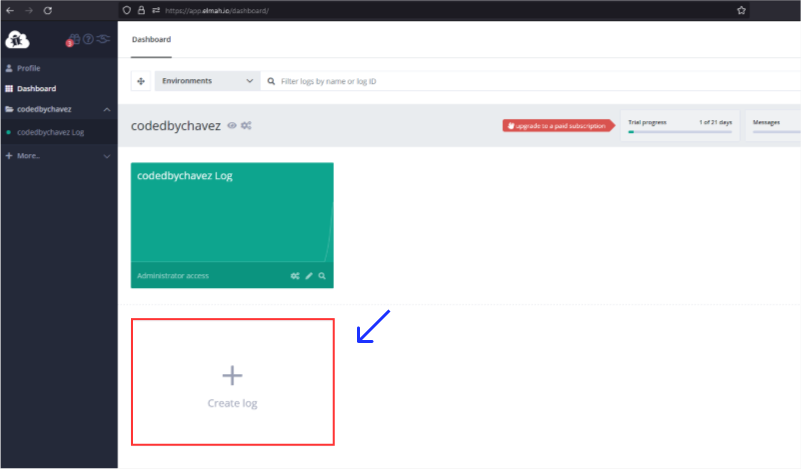This web page dashboard image features various elements and sections, though some text is blurry and difficult to read. In the top left corner, an arrow points to the left. Below this arrow, the left-hand column features a profile icon next to the word "Profile." The subsequent item reads "Dashboard," followed by "Coded by Chavez," all as one phrase. Further along, it displays a section labeled "Coded by Chavez Log," accompanied by a plus sign and the word "More."

To the left, the word "Dashboard" is underlined. Directly beneath this, a dropdown menu is set to "Environments," next to a search bar with a magnifying glass icon containing the placeholder text "Filter logs by name or log ID." Below this section, the text "Coded by Chavez" appears once again. A red rectangle below it contains the text "Update to a paid subscription." Following this is the phrase "Trial Progress, 1 of 21 days," and the word "Messages."

Further down, there is a greenish-blue rectangle with the text "Encoded by Chavez Log" printed on it. Beneath this section, blurry text likely reads "Administrator access." Below this, a white rectangle with a red border appears, highlighted by a blue arrow pointing toward it. Inside this rectangle, there is a plus sign and the phrase "Create Log."